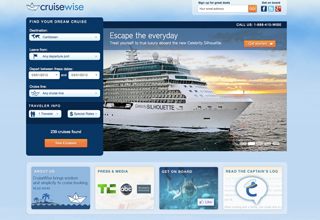This caption describes a detailed screenshot for a website called CruiseWise. 

---

This small screenshot captures the homepage of CruiseWise, easily identifiable by its logo located in the top left corner. The logo features the site name "CruiseWise" alongside a charming doodle of a paper ship, folding up to resemble a cruise liner. The site’s theme primarily incorporates shades of light blue, creating a soothing, nautical ambiance.

On the left-hand side, there's a navigation panel offering practical search options for users to select their travel destination, departure point, travel dates, and other potential preferences. Adjacent to this panel, a vibrant image of a large cruise ship dominates the scene, against a serene sunset background where the sky is a blend of soft blue hues and delicate, wispy clouds. The cruise ship has a name that appears to be “Silhouette,” though the small size of the screenshot renders it difficult to confirm.

At the top of the image, bold text reads “Escape Everyday,” accompanied by smaller text that’s difficult to decipher. On the right side of this text, there’s an orange button with white text, though the exact wording is unclear due to the screenshot’s size. Below the main image and navigation, four distinct tiles are arranged, presumably linking to various sections of the site: an "About Us" section, a "Get On Board" option, a "Read the Captain's Log" tile, and links to media mentions of CruiseWise.